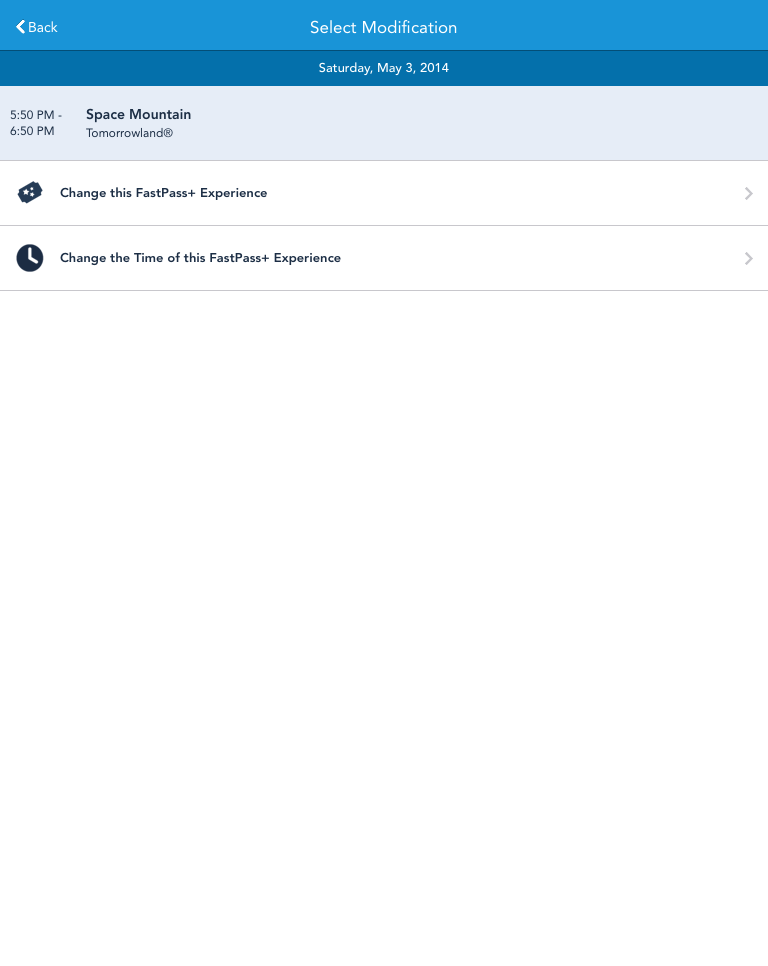The image features a user interface with several layered elements. At the top, there's a light blue rectangular box displaying a white left-pointing arrow labeled "Back." Centrally aligned within this box, the text reads "Select Modification." Beneath it, there's a darker blue rectangle, approximately half the height of the top box, containing the date "Saturday, May 3rd, 2014 (or 2011)"—the text here appears small and somewhat blurry.

Below this, a light gray rectangular box lists specific details including a time, presumably "5:50 PM," followed by the attraction name "Space Mountain." Under this, another time is indicated, possibly around "6 something PM," associated with "Tomorrowland" or a similar term, albeit difficult to read clearly.

Further down, there is a white rectangular box with the option "Change to FastPass Experience" and a right-pointing arrow. Immediately below this is an icon of a clock, accompanied by the text "Change the time of the FastPass Experience," also followed by a right-pointing arrow.